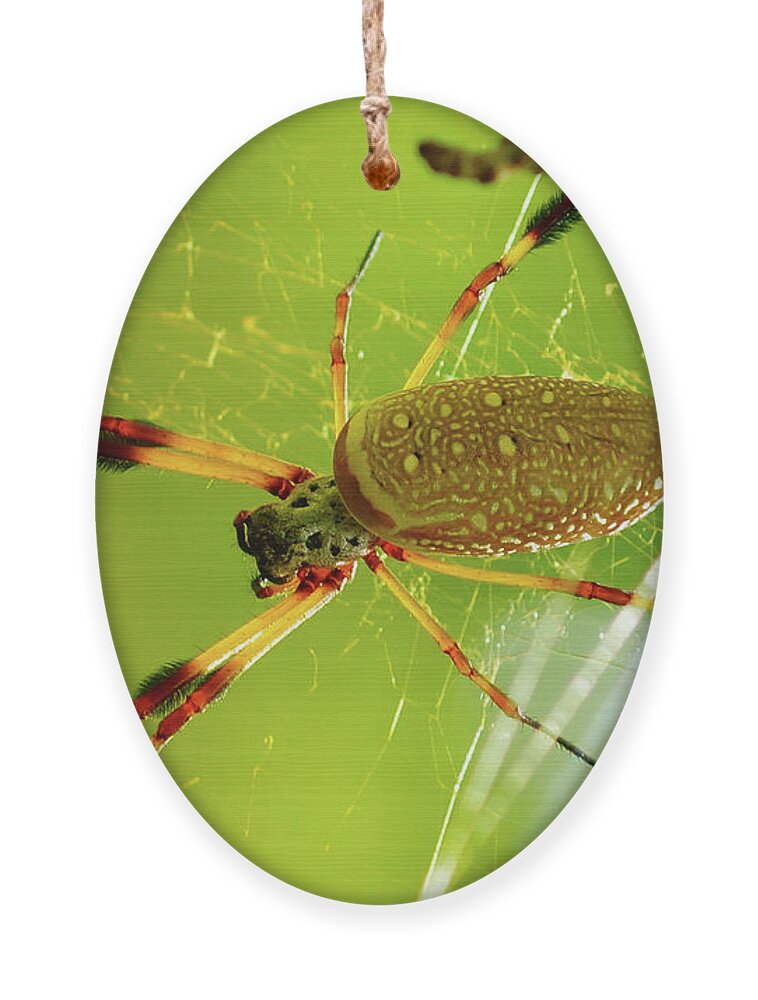The image features an oval-shaped pendant hanging from a string, suggesting it is a piece of jewelry, likely a necklace or keychain. The pendant displays a highly detailed green and yellow spider against a light green background that could be resembling a leaf. The spider has a green body adorned with a speckled brown pattern reminiscent of the texture of a pancake, with lines and dot-like circles. Its legs are light green or yellow, transitioning into a red hue towards the tips, which also have delicate black bristle-like structures. The spider's body occupies much of the pendant, creating a prominent focal point, while the background enhances the intricate design of the insect.